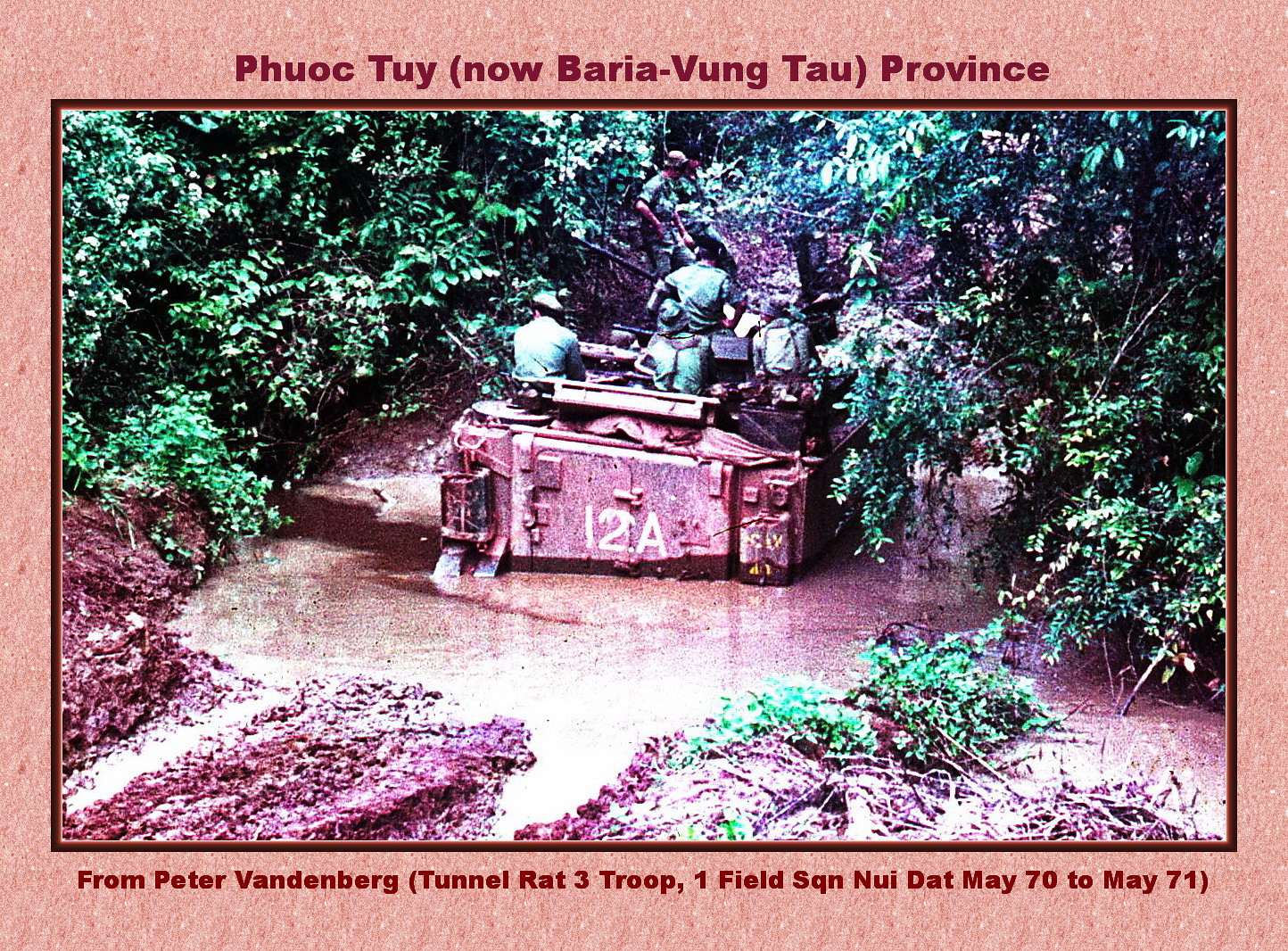This landscape-oriented photograph, set against a peach-coral digital background, is bordered by a thin dark red line creating a frame. At the top of the image, in dark red letters, it reads "Phuoc Toi, now Baria Vung Tau Province," and at the bottom, similarly, it states "From Peter Vandenberg, Tunnel Rat 3 Troop 1 Field SQN Nui Dat May 70 to May 71." The center of the photograph features a tank or amphibious military vehicle navigating through a large muddy puddle or river surrounded by dense jungle vegetation. The vehicle, devoid of a traditional roof, carries four soldiers clad in green military attire and hats, visible atop the vehicle as it makes its way through the rough terrain. The image conveys a vivid scene of military activity during the Vietnam War, emphasizing the challenging conditions faced by the soldiers.